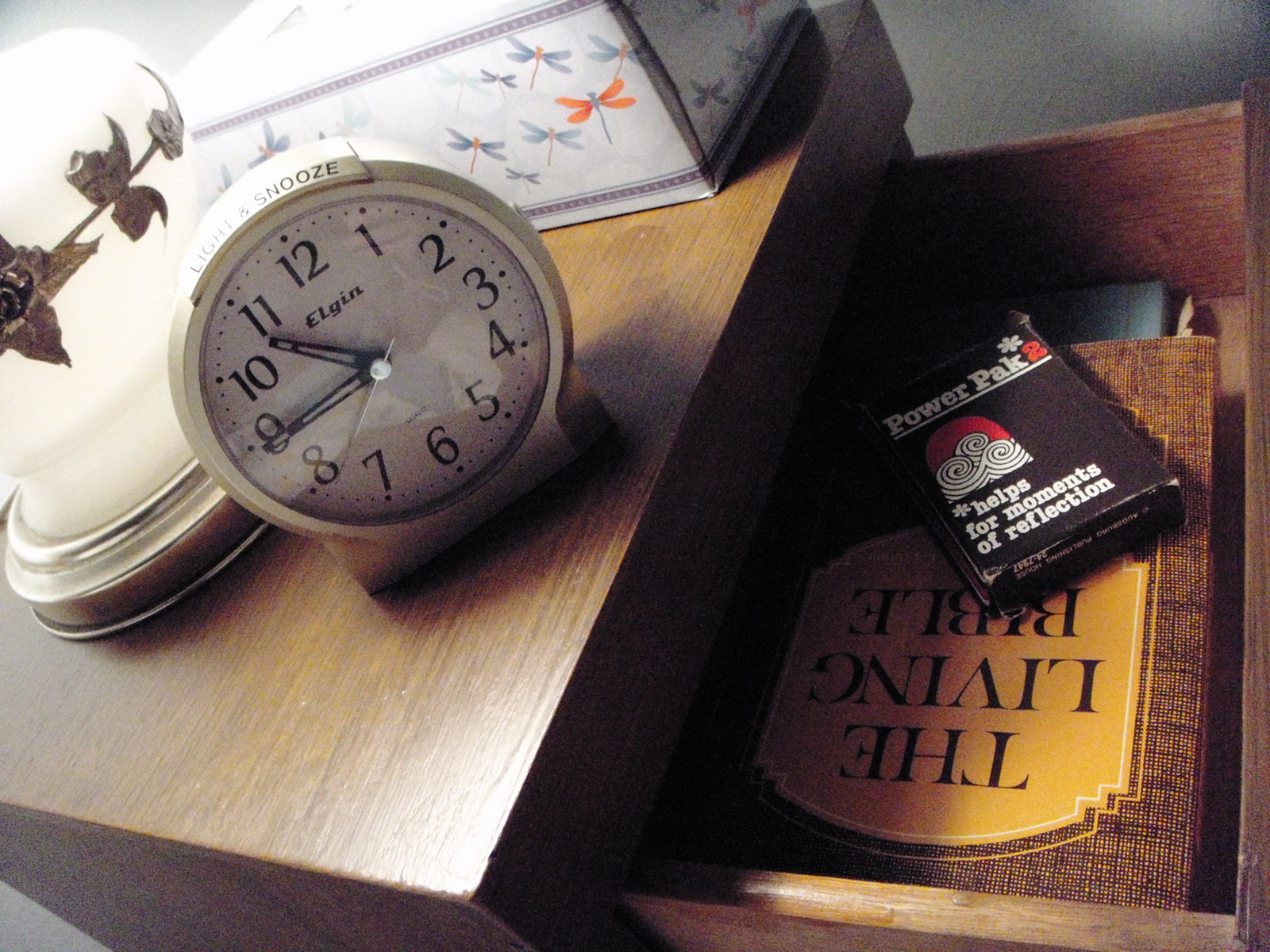The image depicts an angled view of a wooden nightstand with a deep brown oak finish, photographed from the right side. The top drawer of the nightstand is open, revealing its contents. Inside the drawer, there is a brown and tan striped book titled "The Living Bible," which appears upside down from this angle. Resting on top of the Bible is a small black box, similar in size to a deck of cards, labeled "Power Pack 2: Helps for moments of reflection," featuring a red arch with white and black waves. Below the Bible, a blue notebook is partially visible.

On the surface of the nightstand, multiple items are arranged. Centrally placed is a white analog alarm clock with black numbers and hands, including a distinct white second hand. The top of the clock features buttons marked "Light" and "Snooze," with the brand name "Elgin" positioned below the number 12. The clock displays the time as 10:45 PM. Behind the clock, there is a white ceramic lamp with a bronzed metal base adorned with a rose motif winding through its center.

Additionally, on the right side of the nightstand's top, stands a rectangular tissue box decorated with blue colors and dragonfly illustrations, some of which are purple and red.